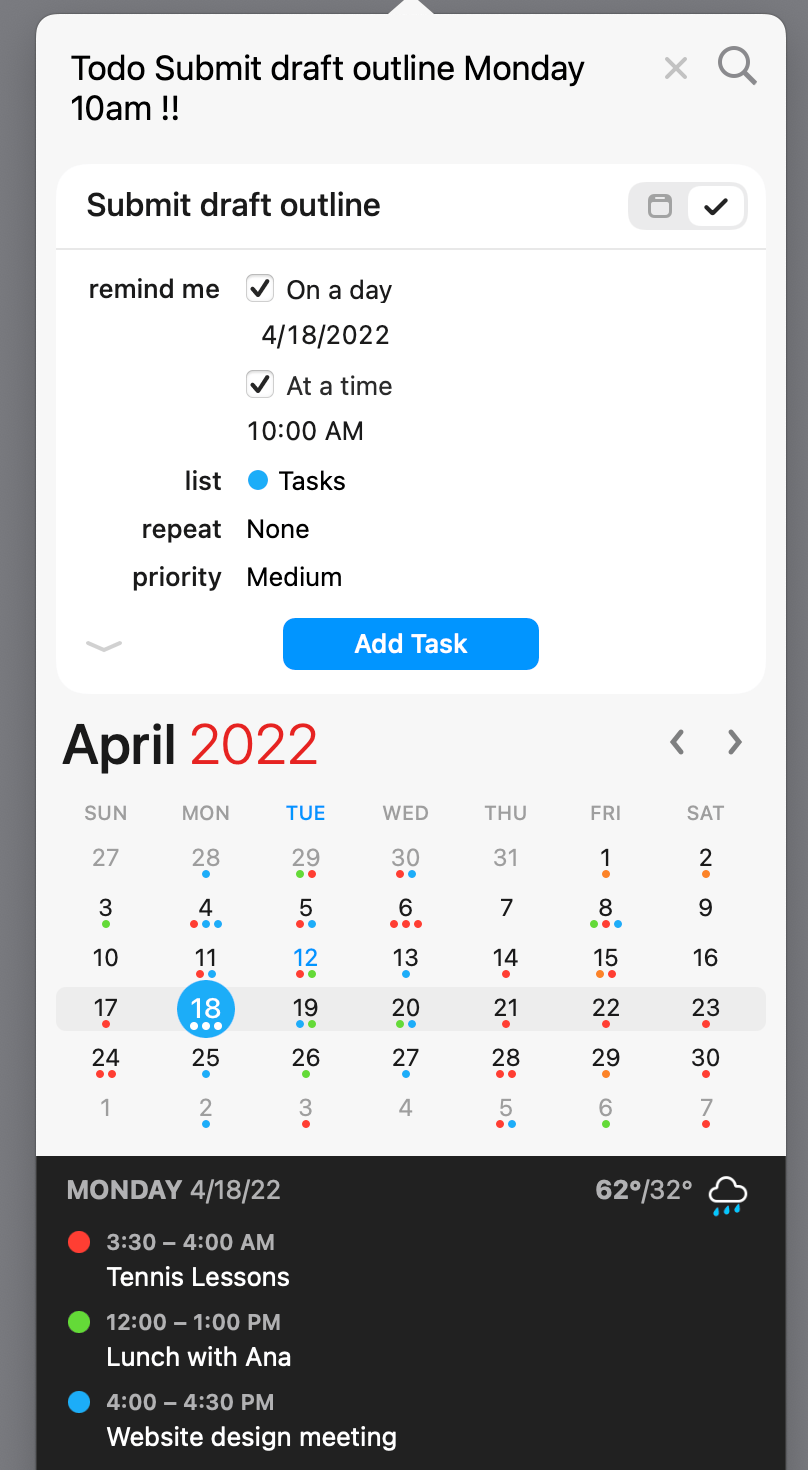This image is a cell phone screenshot framed by a gray border on the left, right, and top edges. At the top, there's a header with the text "To do, submit draft outline Monday 10 a.m.!!" To the right of this text, there is a close button marked with an 'X' and, further to the right, a magnifying glass icon tilted to the left.

Below the header, in a central white section, the text reads "Submit Draft Outline." Adjacent to it, there is a gray and white selection box: the left side in gray with a square icon and the right side in white with a black checkmark.

The subsequent text indicates the reminder details: "Remind me on a day 4-18-2022 at a time 10 a.m. List tasks, repeat, none, priority, medium." There are checkboxes next to "on a day" and "at a time," both of which are checked. Centrally located is a blue rectangular button with white text that says "Add Task."

Below this section is an April 2022 calendar. "2022" is displayed in red font at the bottom of the page. Against a black background, it reads "Monday 4-18-22," with the temperature "62°F / 32°F" and a rain cloud icon on the far right.

Further down on the left, event details appear as colored dots: a red dot for "3:30-4 a.m. Tennis Lessons," a green dot for "12-1 p.m. Lunch with Anna," and a blue dot for "4-4:30 p.m. Website Design Meeting."